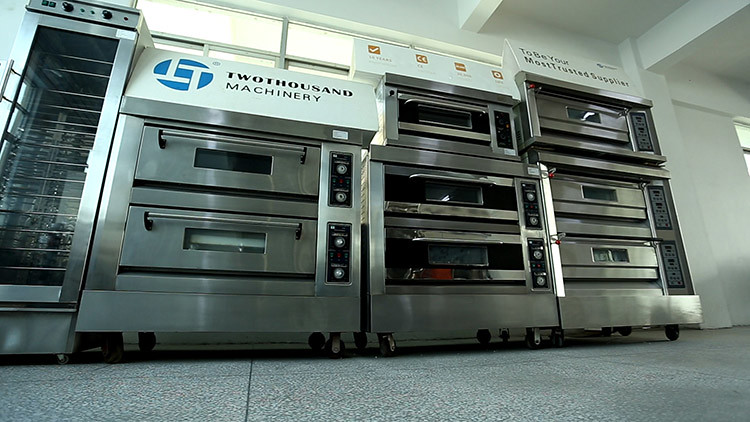The image features a display of industrial ovens in a showroom or commercial facility. There are a total of eight brand-new, stainless steel ovens with black accents, arranged in stacks of three, three, and two from left to right. These ovens seem to be designed for commercial use, likely for restaurants. Above the two stacked ovens on the far right, a sign reads "2000 Machinery" with a blue emblem featuring two T's, one inverted. To the right of this sign, another readable sign states, "To Be Your Most Trusted Supplier." Each of these ovens is mounted on wheels, enhancing their commercial appeal as portable units. The setting includes a light gray tiled floor and white walls, with columns visible across the ceiling. On the far left, there's a tall stainless steel appliance with a glass door, possibly a rotisserie, adding to the collection of commercial kitchen equipment. A large window is situated just above the "2000 Machinery" sign, allowing natural light to illuminate the display. The viewpoint of the image is diagonal, taken from a lower angle, which provides a comprehensive view of the equipment arrangement.